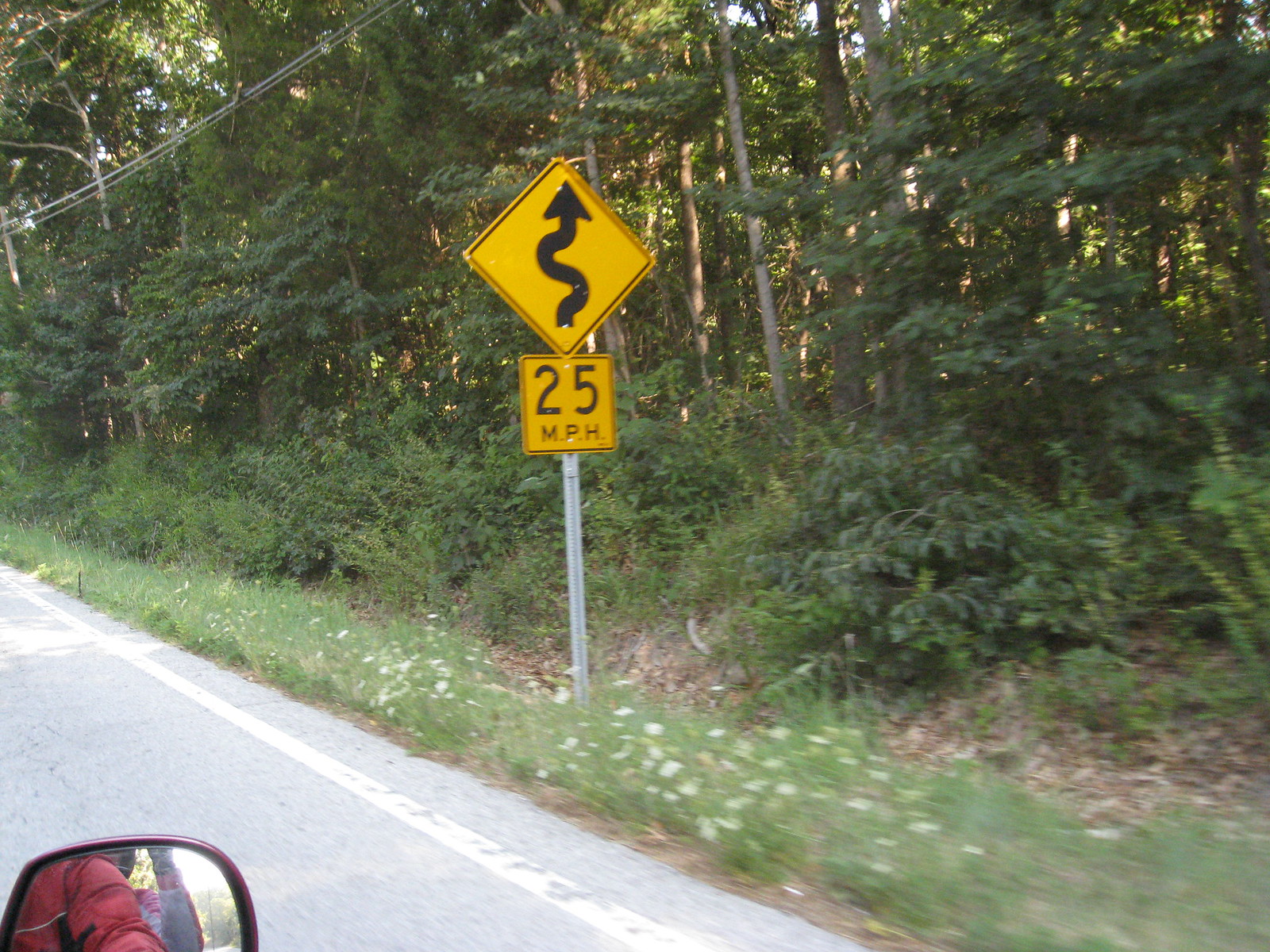A vibrant photo captured from within a car, featuring the side mirror in the bottom left corner, reflecting the arm and shoulder of the driver clad in a red shirt. The partially visible shoulder and sleeve add a subtle human element to the scene. The photograph unveils a picturesque view outside the car window, starting with a strip of road displaying a jagged white line along its edge, transitioning into a patch of wild, unkempt grass adorned with scattered flowers. A prominent road sign indicating a speed limit of 25 miles per hour and a curving road ahead stands amidst the greenery. The backdrop is bustling with a dense array of trees, through which diffused sunlight glimmers softly. In the upper left corner, an electric wire stretches across, adding an element of human presence to this tranquil, natural setting.